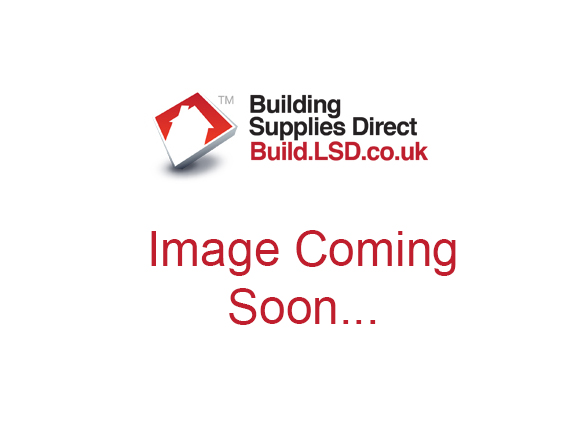The image features a minimalistic ad set against an all-white background that seamlessly fades into the computer screen's background. At the top in bold black letters, it reads "Building Supplies Direct." Below this primary title, in a striking red font, is the URL "build.lsd.co.uk". To the left of the text, there is a trademark symbol (TM) beside a red square logo, which is tilted to rest on its bottom left corner like a diamond. The logo contains a white house icon with a chimney. Below all of this, in large sans-serif red letters, are the words "IMAGE COMING SOON...". The ad's clean design emphasizes the anticipation of content on this new building supplies website, with key colors being black, red, and grey.